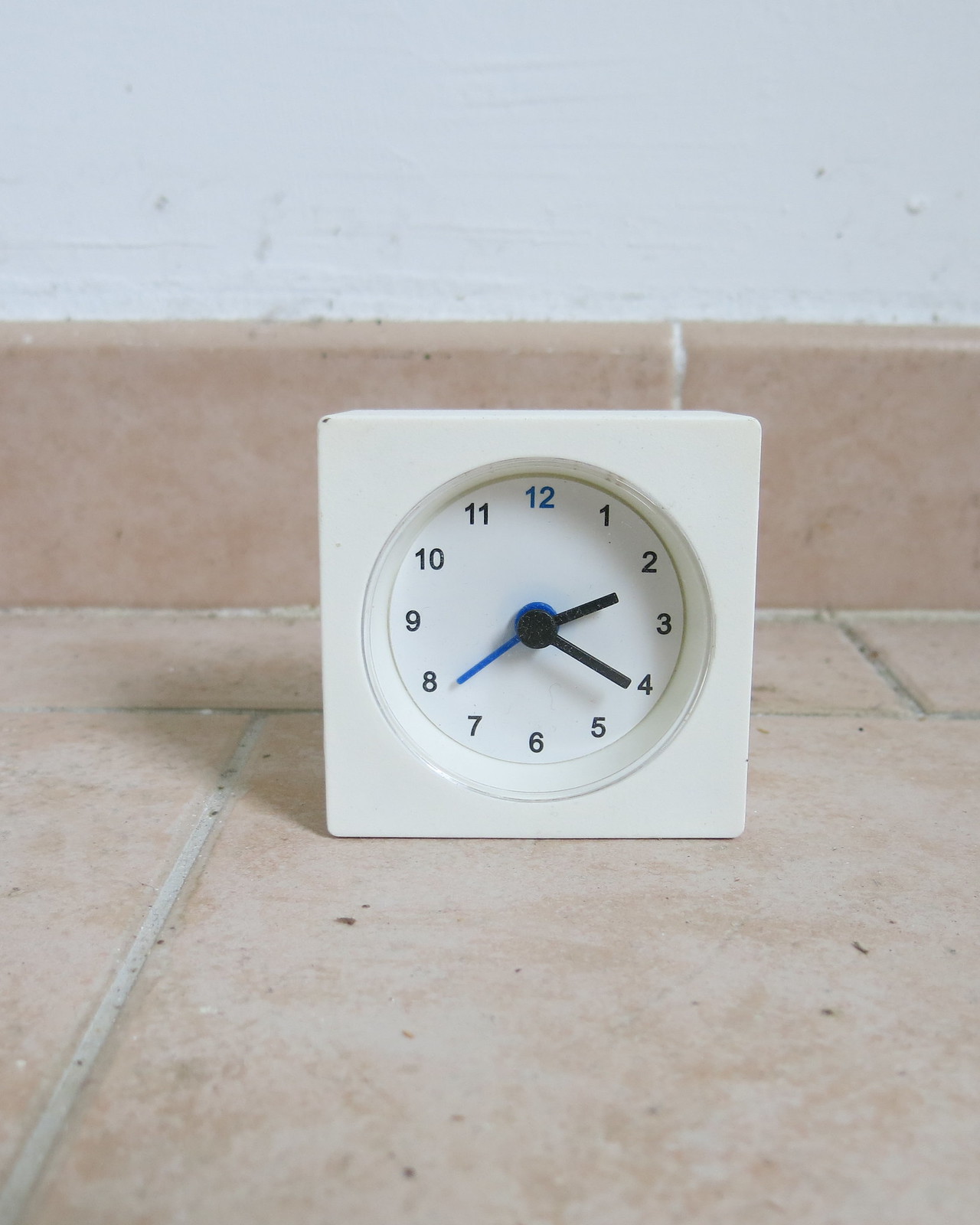A sleek, modern box clock encased in a clear, white frame features a minimalist design with a traditional watch face displaying Arabic numerals from 1 to 12. The time reads approximately 2:21 and 38 seconds, as indicated by the hour, minute, and second hands. The scene is illuminated by artificial lighting, adding a contemporary touch to the setting.